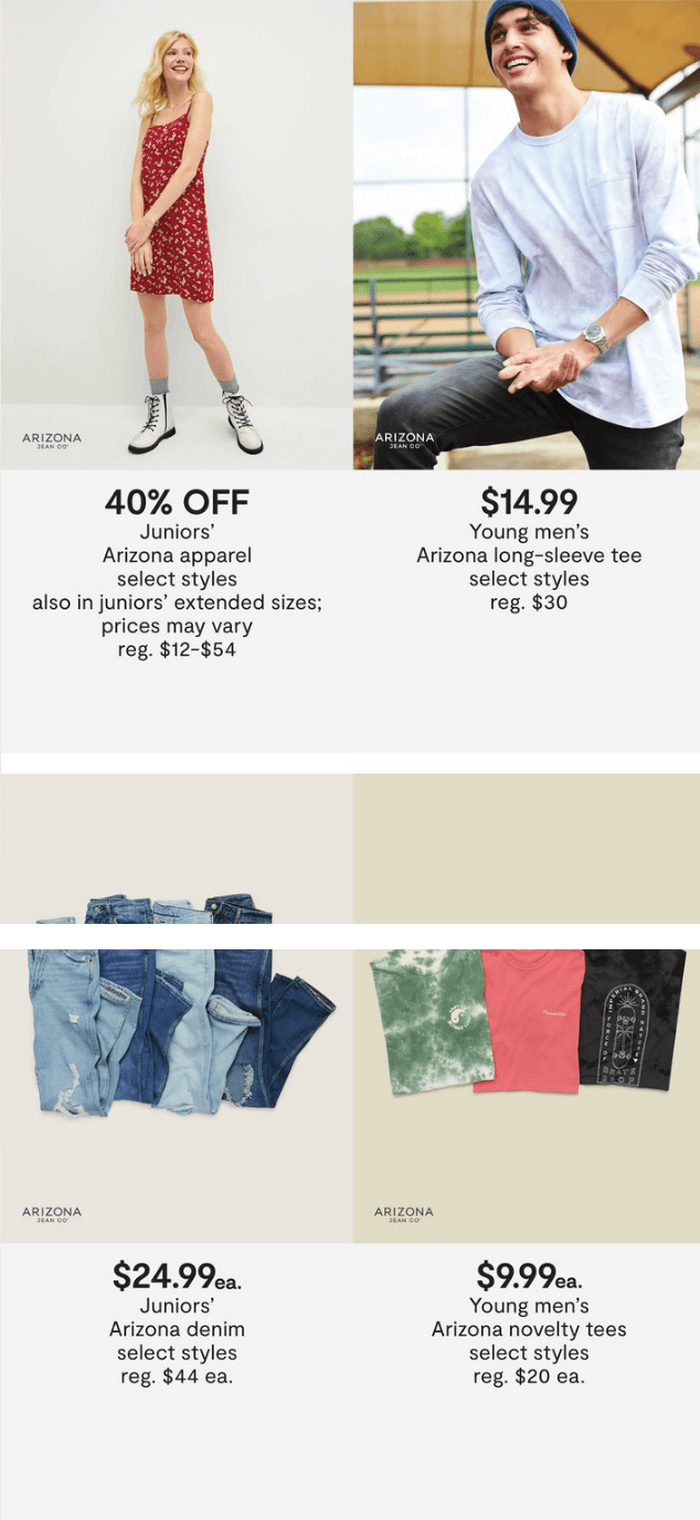In the upper left-hand corner of this screenshot, there is a square image with a light gray background featuring a woman in a red printed dress. Adjacent to this, on the right, is another square image of a young man wearing a long-sleeve white t-shirt and black jeans. Centered below the woman's image, in bold black text, is a highlighted discount message: "40% OFF" which is larger than the surrounding text. Below this, in a smaller font, it reads: "Juniors, Arizona apparel, select styles, also in juniors extended sizes. Prices may vary. R.E.G. $12-$54."

Underneath the young man's image, there is the price "$14.99" followed by the description: "Young men's Arizona long-sleeve tee, select styles, R.E.G. $30". The screen is visually divided by a white rectangular line, creating almost a split view.

In the lower left-hand square, an image of jeans is displayed with a price tag of "$24.99 each" and the description: "Juniors Arizona denim, select styles, R.E.G. $44 each." In the lower right-hand square, there are three t-shirts with a price tag of "$9.99 EA" followed by: "Young men's Arizona novelty tees, select styles, R.E.G. $20 EA."